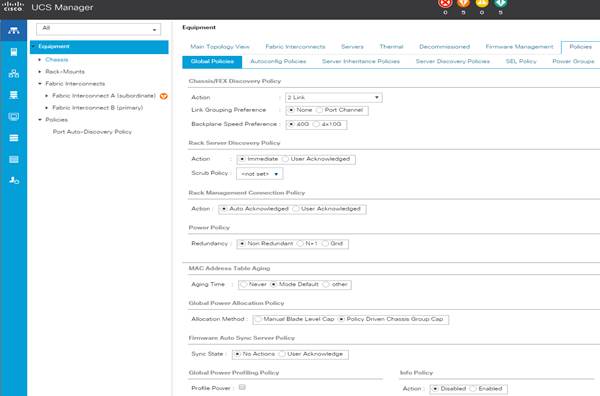The image is a screenshot of a computer interface displaying the UCS Manager software, as indicated by the label "UCS Manager" in the upper left corner. Below this label, a prominent black navigation bar spans the width of the screen with various icons and symbols aligned on the right side. Among the symbols are four circular indicators: a red circle with an "X," an orange circle with a triangular symbol, a yellow circle, and a green circle.

Beneath the navigation bar, a list is visible. Although the exact selection is unclear, it appears that the top item in this list has been clicked. To the right of the list, there's a column labeled "Equipment" highlighted in blue. Above this, another section also labeled "Equipment" is visible, and text to the right suggests that another item has been selected, possibly reading "Old School."

The main content area is filled with several rows of small, black text separated by lines, making the information difficult to read due to the text size.